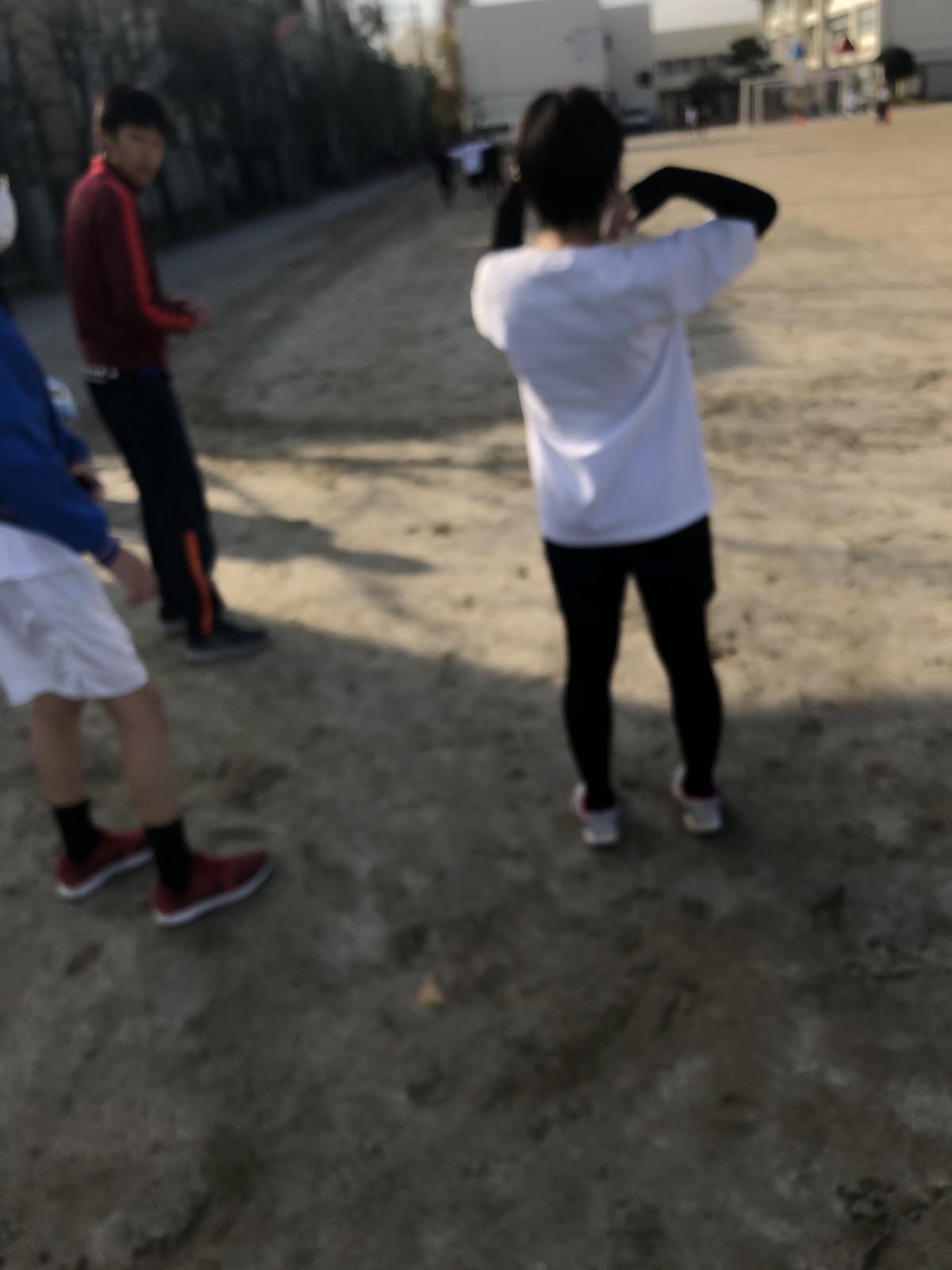This blurry outdoor photograph captures three young boys, around ten years old, standing on a dirt lot with a tall wall on the left side and a distant building visible at the top right. In the foreground, partially visible on the left, there's a boy wearing a blue long-sleeve shirt, white shorts, black socks, and red and white shoes. Facing the camera, another boy in front of him dons a long-sleeve purple shirt with a red stripe, black pants with a red stripe, and gray shoes. To the right, the third boy wears a short-sleeve white shirt over a long black sleeve shirt, black sweatpants, and white shoes. The image is quite out of focus, with the boys' sneakers being the most identifiable part of their outfits, and only portions of their legs and torsos discernable as they all stand together on the dirt surface.